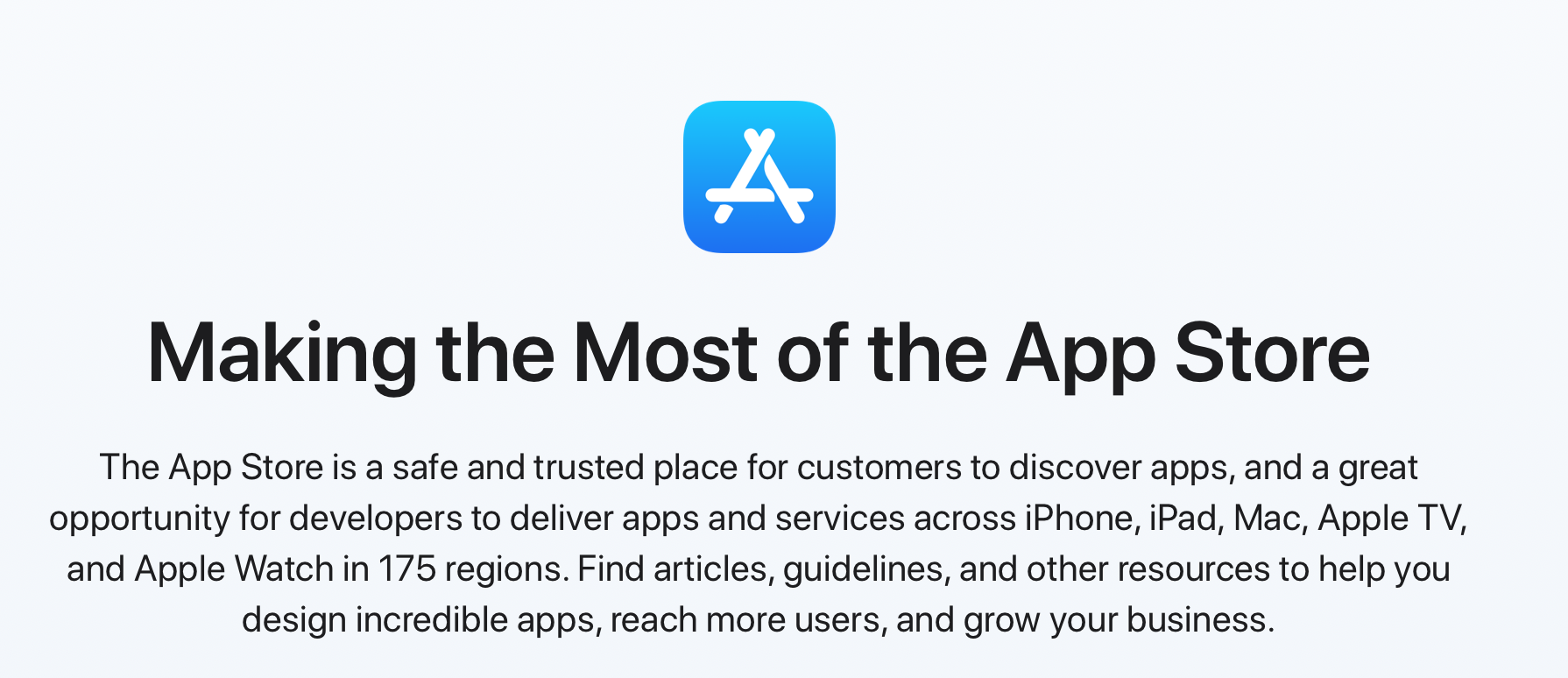The image appears to be a banner, possibly a screenshot from an Apple web page, with a light gray background. Centrally positioned in the upper section is the Apple App Store logo, characterized by a blue square with rounded corners, shading from a darker hue at the bottom to a slightly lighter shade at the top. The logo prominently features a stylized "A" composed of three white popsicle stick-like shapes.

Directly beneath the logo, bold black text reads: "Making the most of the App Store." Below this, in smaller black text, the caption elaborates: "The App Store is a safe and trusted place for customers to discover apps and a great opportunity for developers to deliver apps and services across iPhone, iPad, iMac, Apple TV, and Apple Watch in 175 regions. Find articles, guidelines, and other resources to help you design incredible apps, reach more users, and grow your business."